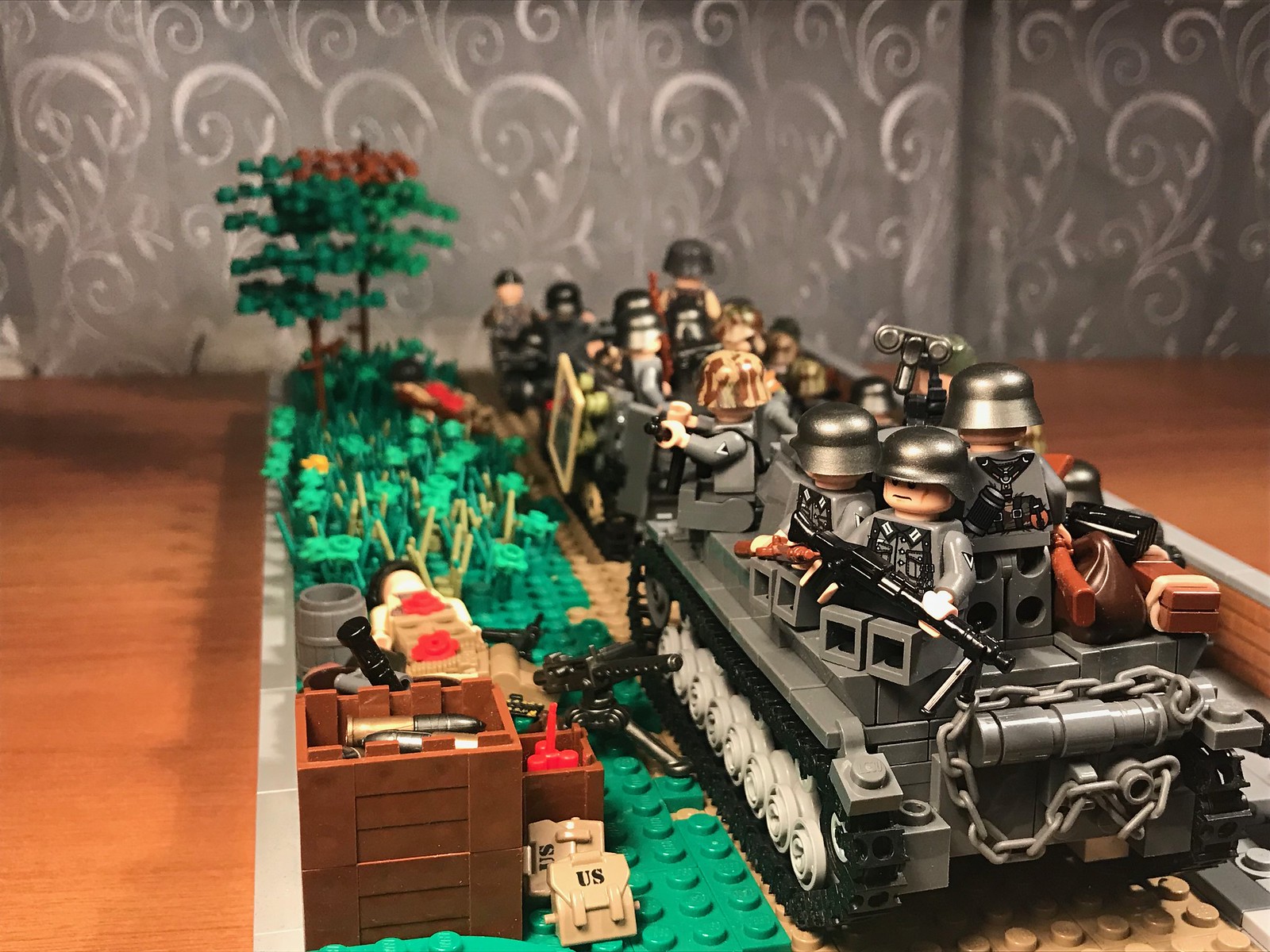This image depicts an extensive and intricate Lego scene set on a brown table with a backdrop that appears to be a gray drape adorned with lighter gray, possibly paisley, plant designs. The Lego construction prominently features several tanks and soldiers. On the right side, there is a well-defined tank with Lego soldiers holding black rifles and sporting silver helmets and gray bodies. Some of the soldiers have camouflage brown helmets. Behind this tank, another tank is visible with more armed soldiers. In the middle left section, there are Lego containers holding bullets, and a small fort structure is built nearby. The foreground is adorned with a grassy area, tiny bushes, and two Lego trees with green and red leaves. Scattered on the scene are also US vests, all meticulously crafted from Legos. The setting extends from the lower right to the left, filling the entire square image. The floor beneath this elaborate setup consists of wooden tiles.